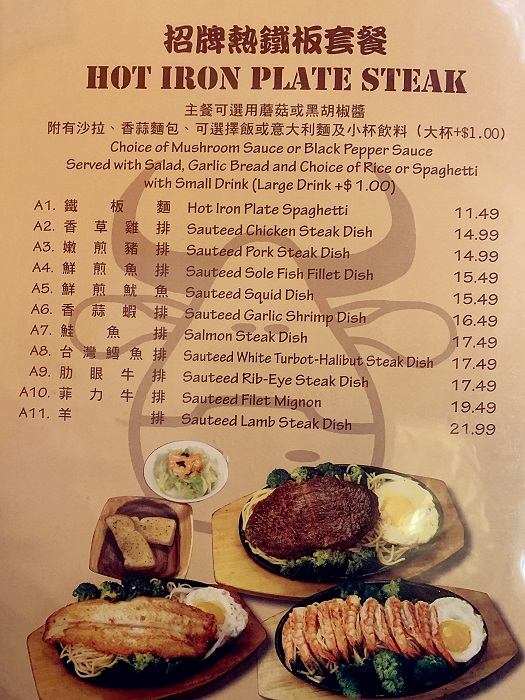The image showcases a bilingual menu featuring both English and an Asian language, likely Japanese or Chinese. The menu is presented in portrait orientation with a predominantly brown color scheme. The background is a light brown shade, complemented by dark brown or orange text. A watermark of a cow with dark horns, beady black eyes, side-facing ears, and a snout is subtly visible in the backdrop.

At the top of the menu, there is a header in bold dark brown Asian characters. Below this, in large bold capital letters, it reads "HOT IRON PLATE STEAK." Further down, two additional lines in the foreign language are followed by English text detailing the food options: "Choice of mushroom sauce or black pepper sauce. Serve with salad, garlic bread, and choice of rice or spaghetti. With small drink, large drink, plus one dollar."

The menu lists items labeled A1 through A11, with prices ranging from $11.49 to $21.99. Some highlighted dishes include Hot Iron Plate Spaghetti, Sautéed Chicken Steak Dish, Sautéed Pork Steak Dish, Sautéed Salt Fish Filet Dish, and the most expensive option, Sautéed Lamb Steak Dish.